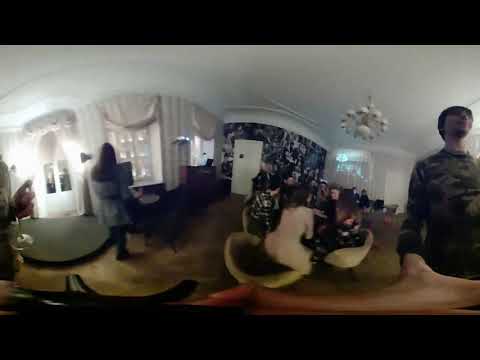This wide-angle photo captures an indoor living room scene with several individuals and distinct features. On the left side of the room stands a woman with long hair, her back turned to the camera. She is dressed in gray and wears jeans with a long shirt extending to her knees. In the center of the image, another woman, clad in a white dress, is seated on a bench or chair. To her right, a man in a gray sweater or possibly a camouflage long-sleeve shirt stands facing the white wall, which features a set of lights and a white chandelier hanging from the ceiling. He appears young, potentially a teenager, with a mop-top haircut. The room has a brown floor, and on the far left side, there's a white door with two windows that are slightly illuminated, suggesting it might be evening. The overall room color scheme includes white walls and a ceiling, with a section of the wall adorned with blue floral wallpaper near the white door. The lighting within the room is somewhat dim, creating a cozy yet slightly shadowed ambiance.